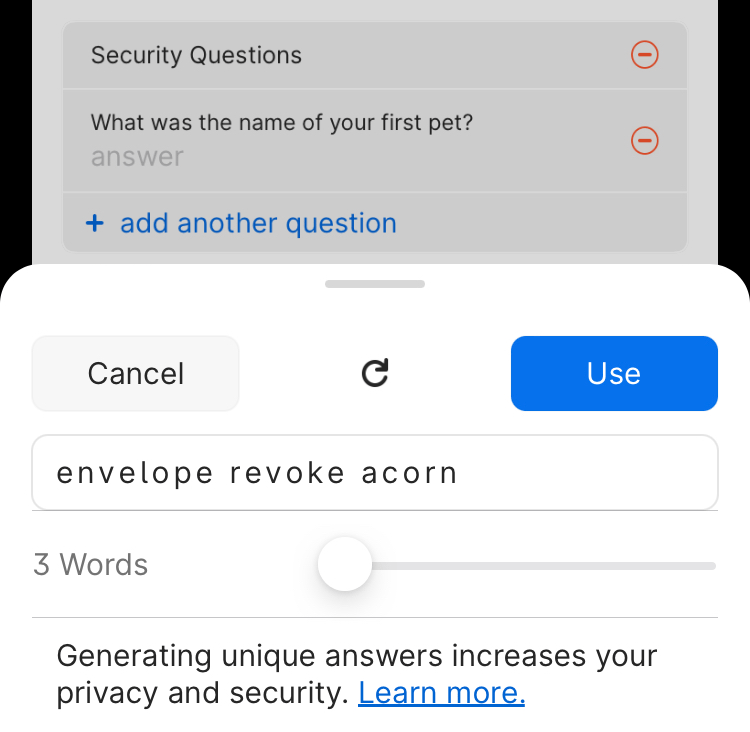This image, captured from a digital screen which could be a phone or a computer, displays a section for security questions. At the top, in a gray box with white text, it says "Security Questions." To the right of this title, there is a red minus symbol encased within a white circle, which itself is outlined by a red border, indicating an option to remove this question.

The first listed security question reads, "What was the name of your first pet?" Directly beneath this question, in gray print, is the word "Answer," along with the same red minus symbol encased within a white circle, and a red border as seen earlier. Below this is a blue-colored prompt with a white plus symbol and the text "Add Another Question," allowing the user to add additional security questions for enhanced privacy.

Further down, on the left-hand side of the screen, is a "Cancel" button. In the middle, there is a refresh arrow icon. To the right, a blue rectangular button with the word "Use" written in white text is visible. 

Below this section, three words— "envelope," "revoke," and "acorn"—are displayed along with a slider interface, suggesting selectable options for additional security measures. At the bottom, the text "Generating unique answers increases your privacy and security," followed by a "Learn more" link, offers additional information on enhancing user privacy.